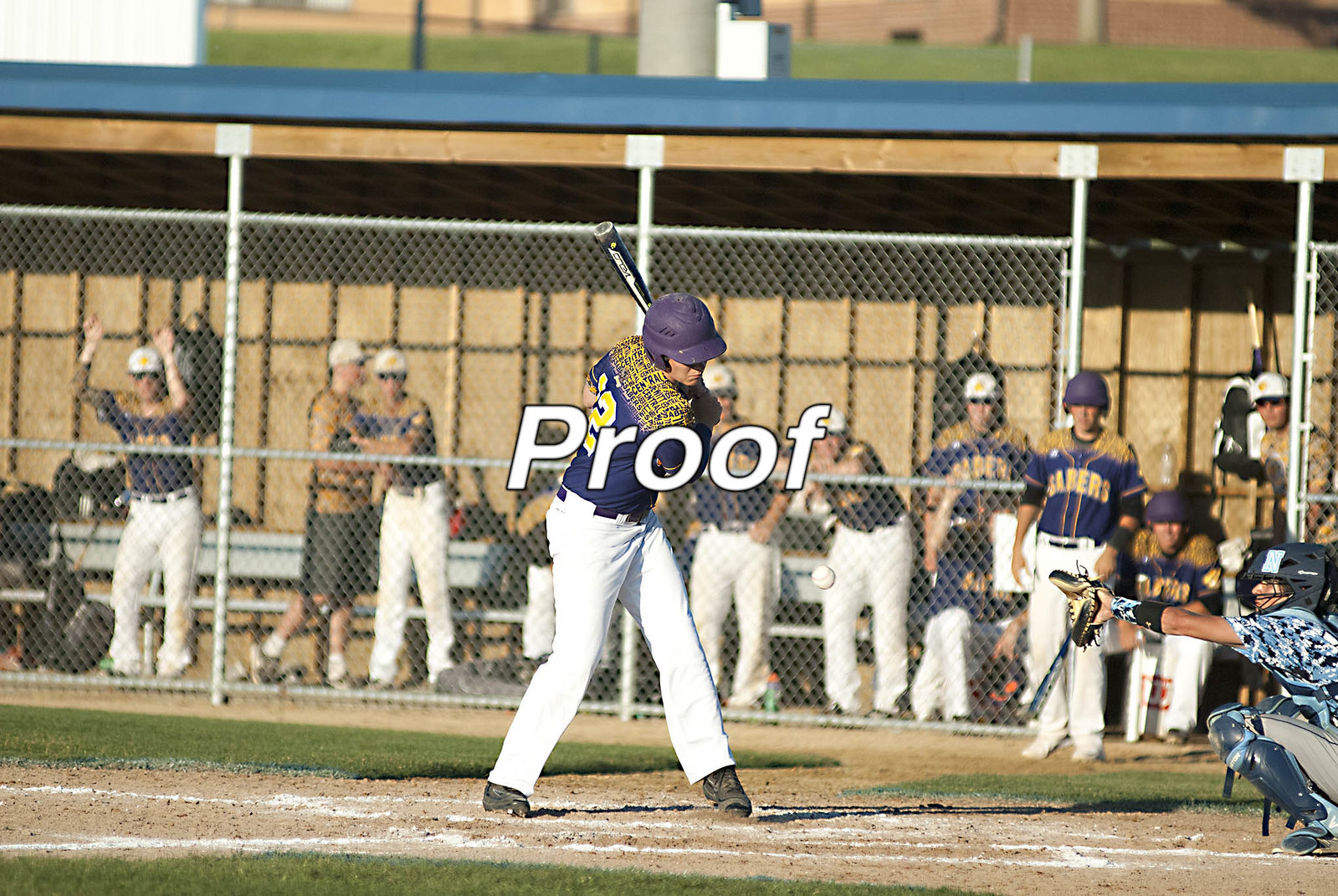This is a detailed proof photograph capturing an action shot of a baseball game in progress. In the forefront, the batter, dressed in a dark blue jersey with yellow lettering and shoulder accents, white pants, and a purple helmet, is poised to swing at an incoming ball. His bat is ready, and he appears to be focused on the ball approaching him mid-air. The number on the back of his jersey is partially visible, showing a '2'. Standing behind the batter, the catcher, in full gear with an outstretched mitt, awaits the pitch. The umpire, dressed in a blue shirt with matching leg guards and holding a mitt, is also positioned behind the catcher. In the background, other players in matching uniforms of white pants and dark blue jerseys with purple helmets are visible in the dugout area behind a chain link fence. The word "PROOF" is prominently displayed in white letters across the top of the image, indicating the nature of the photograph. The scene exudes a professional atmosphere, vividly capturing the anticipation and intensity of the moment.